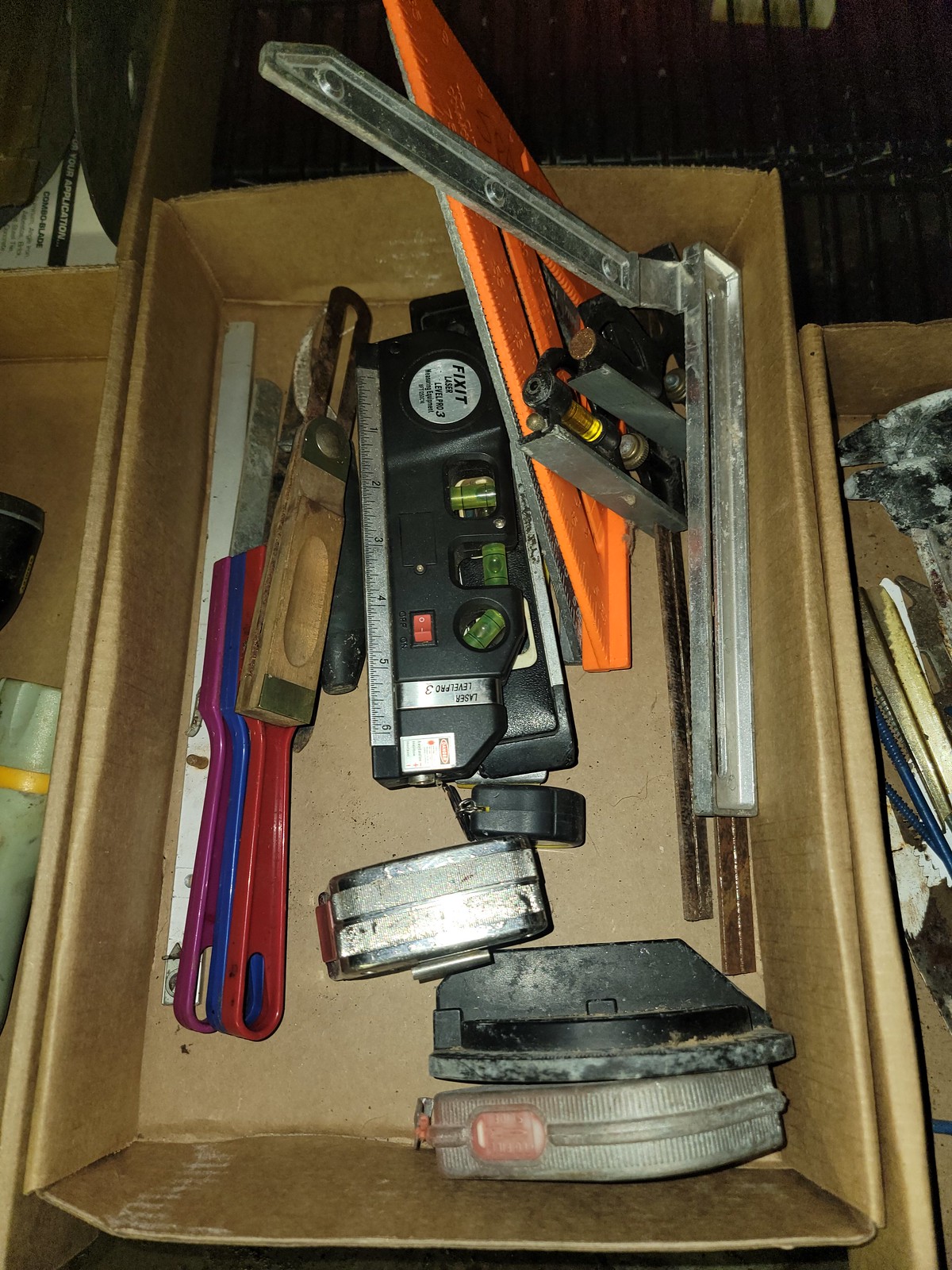This photograph captures the interior of a well-worn cardboard box filled with an assortment of vintage carpenter’s tools, exhibiting signs of heavy use. Central to the image is an older, small, retractable tape measure in a compact form. Surrounding it are various measuring and leveling tools, including a string line for marking and multiple types of bubble levels and corner levels. Several scraping knives and plastic scraping blades can be seen, alongside a unique folding metal tool that forms an L-shape. Diverse tools with colorful plastic handles—red, blue, purple, and green—are also noticeable, although their specific functions are unclear. Among the tools is a larger black unit combining a tape measure and levels, indicative of an advanced measuring device. Adding to the assortment, a rectangular wooden-handled hand tool with a protruding metal section lies nestled inside. Flanking the main box are additional cardboard boxes; one to the left contains a black flashlight, while the one on the right holds more unidentified items, contributing to the trove of utilitarian tools within the main box.